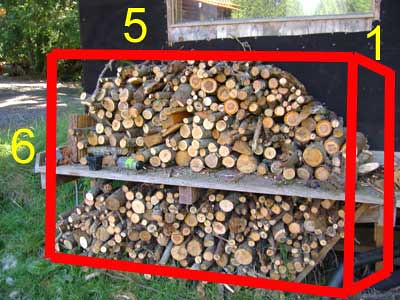The image is a small, low-resolution, digitally altered color photograph depicting an outdoor scene featuring unmanaged grass with scattered leaves or stones in the foreground. Central to the image is a black-wall backdrop against which stands an organized shelving unit filled with chopped firewood. The firewood is arranged in two distinct piles: one atop the shelf and the other beneath it, each log displaying its cross-section towards the viewer. Enhancements include a red rectangular outline digitally superimposed around the wood, suggesting construction guidance for a protective enclosure; the box’s sides are marked with yellow numbers, with "6" on the left, "5" on the top left, and "1" on the top right. In the background, there’s a grey window visible in the upper right corner.